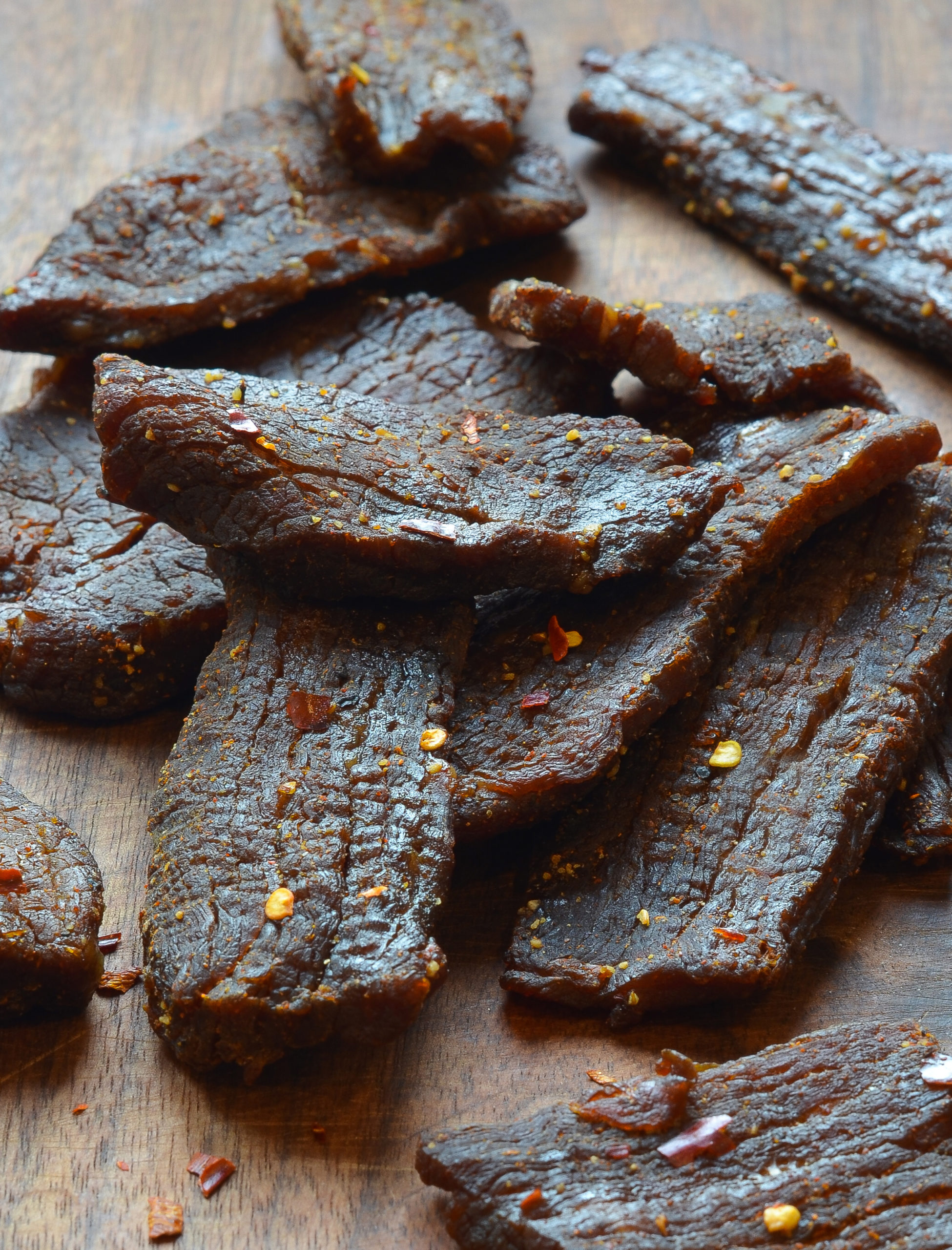The photograph captures a vertical, rectangular image of several strips of beef jerky laid out on a medium brown, slightly distressed wooden surface, possibly a charcuterie board or cutting board. The beef jerky, characterized by its deep brown color and dry, cracked texture, is encrusted with an assortment of spices, including visible red chili pepper flakes and other orange and cream-colored spice specks. The pieces of jerky, varying in length, are arranged haphazardly on top of one another, showcasing their striated surfaces—a result of the dehydration process. The scene conveys a rustic, appetizing presentation of this popular dried meat snack.